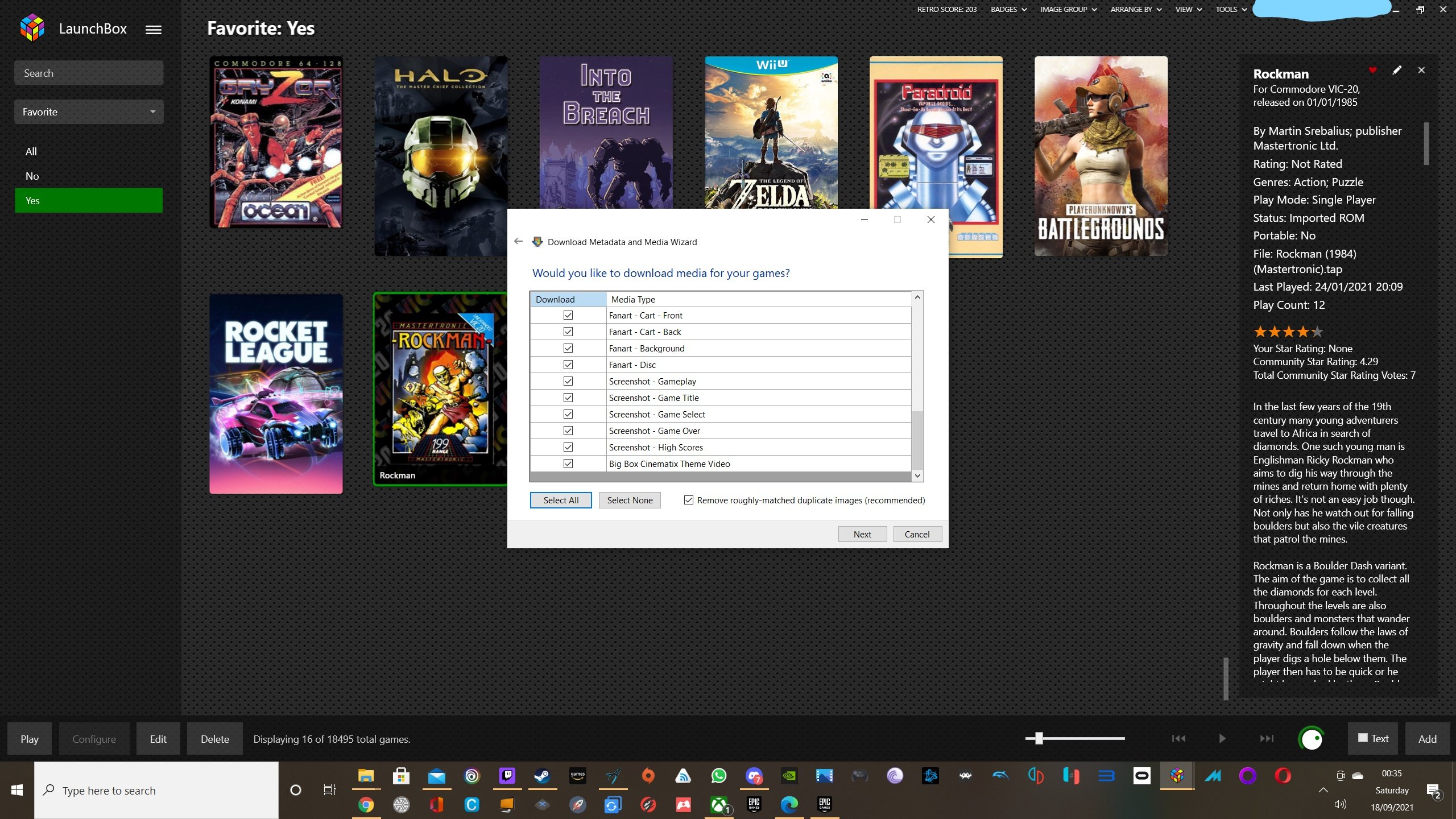This color image captures a website with a dark, predominantly black background. Centrally featured is a row of video game thumbnails or covers, showcasing titles like Halo, Into the Breach, Zelda, Paranoid, Rocket League, and PlayerUnknown's Battlegrounds, among others. 

In the center of the webpage is a dialog box titled "Download Metadata and Media Wizard." The text in blue asks, "Would you like to download media for your games?" Below this prompt is a two-column table. The leftmost column is labeled "Download" and consists of a series of checkboxes, all of which are checked in this particular instance. The second column is headed "Media Type" and lists various types of media such as Fan Art, Screenshot, Big Box, Cinematics, and Theme Video.

Below the table, there are options labeled "Select All," "Select None," and "Remove Roughly Matched Duplicate Images" (the last option being recommended). At the bottom of the dialog box, there are two actionable buttons: "Next" and "Cancel."